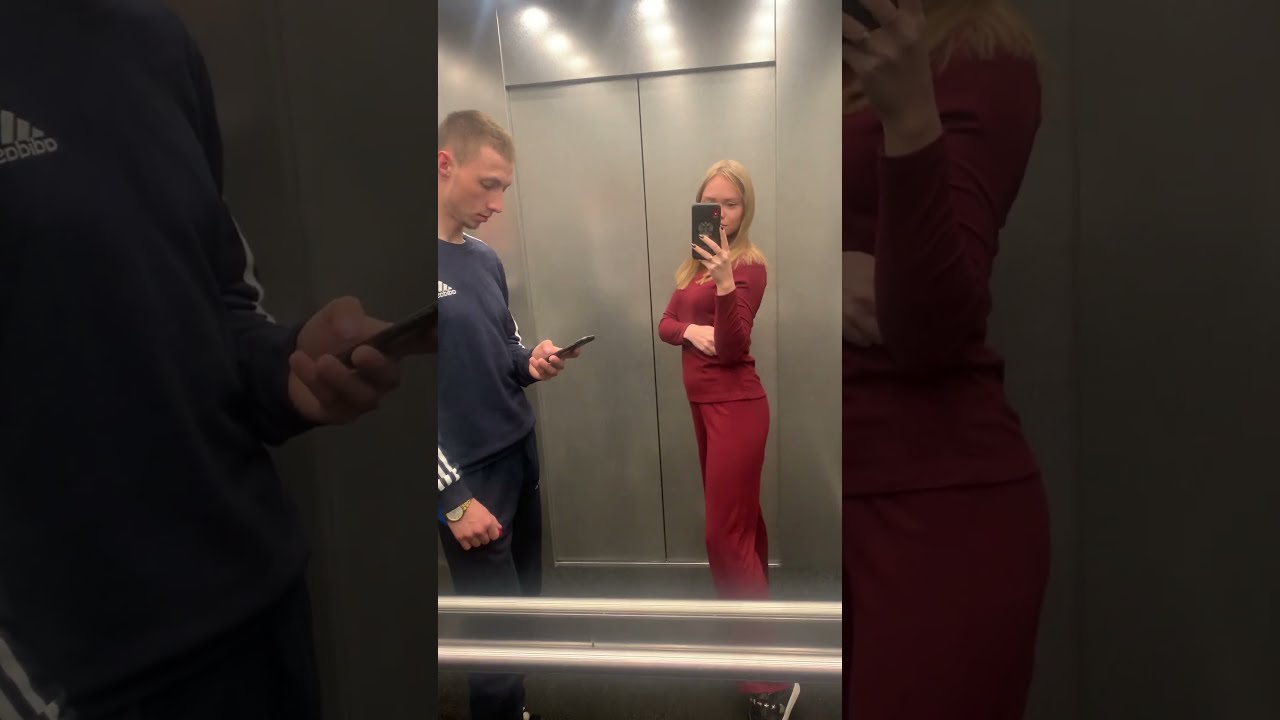In this well-lit indoor image taken in an elevator, we can see two people centered in the frame. On the left is a young man with short hair and a pencil goatee, dressed in a blue Adidas tracksuit. He is focused on his phone, with a gold watch visible peeking out from his sleeve. On the right, a woman with golden hair is wearing a red outfit consisting of a long sleeve shirt and pants. She is taking a selfie using her phone, holding it up to the mirror behind them. The elevator's interior is characterized by its silver steel walls and three rows of ceiling lights that are reflected brightly in the mirror. A silver handrail runs along the right side, and the closed elevator doors can be seen in the background. The overall scene is bathed in a mix of blue, white, silver, gray, red, and yellow hues.